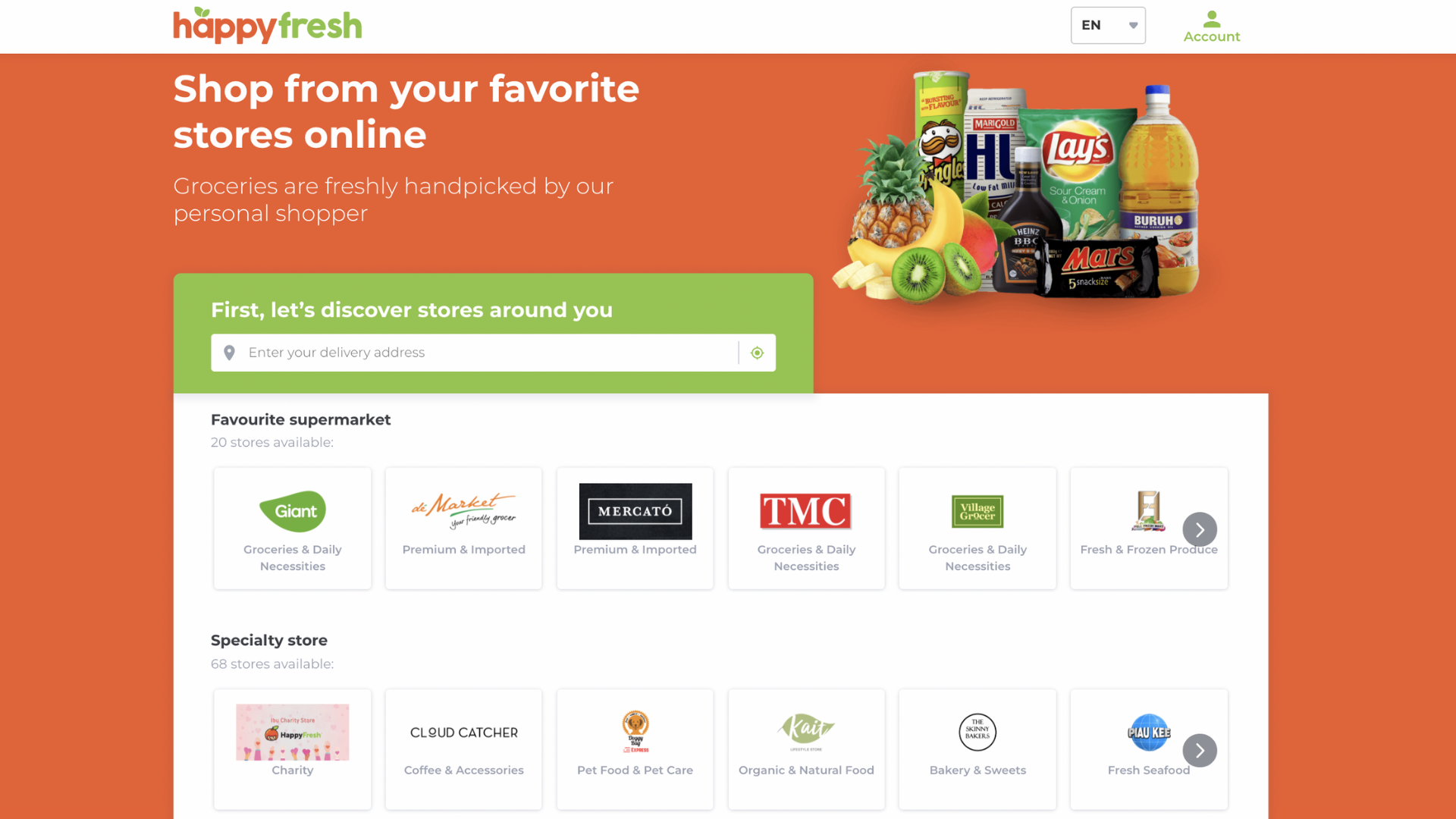This image showcases a webpage from the Happy Fresh website. The Happy Fresh logo is prominently displayed at the top, with "Happy" in orange and "Fresh" in green, and a small green mark above the "A" in "Happy." On the right-hand side, there are options for "Account," represented by an icon of a person, and a language selection menu, indicated by "EN" with a downward arrow for English.

The main background color of the email is a vibrant orange. At the top, a message reads "Shop from your favorite stores online," followed by a search bar that invites users to "First, let's discover the stores around you."

The central image features a diverse array of food items from various brands. The assortment includes fruit such as pineapple, banana, and two kiwis, alongside snacks like Pringles, Lay's chips, and a Mars bar.

Below this image, there is a section showcasing favorite supermarkets, organized into two rows with six icons each, totaling twelve supermarkets.